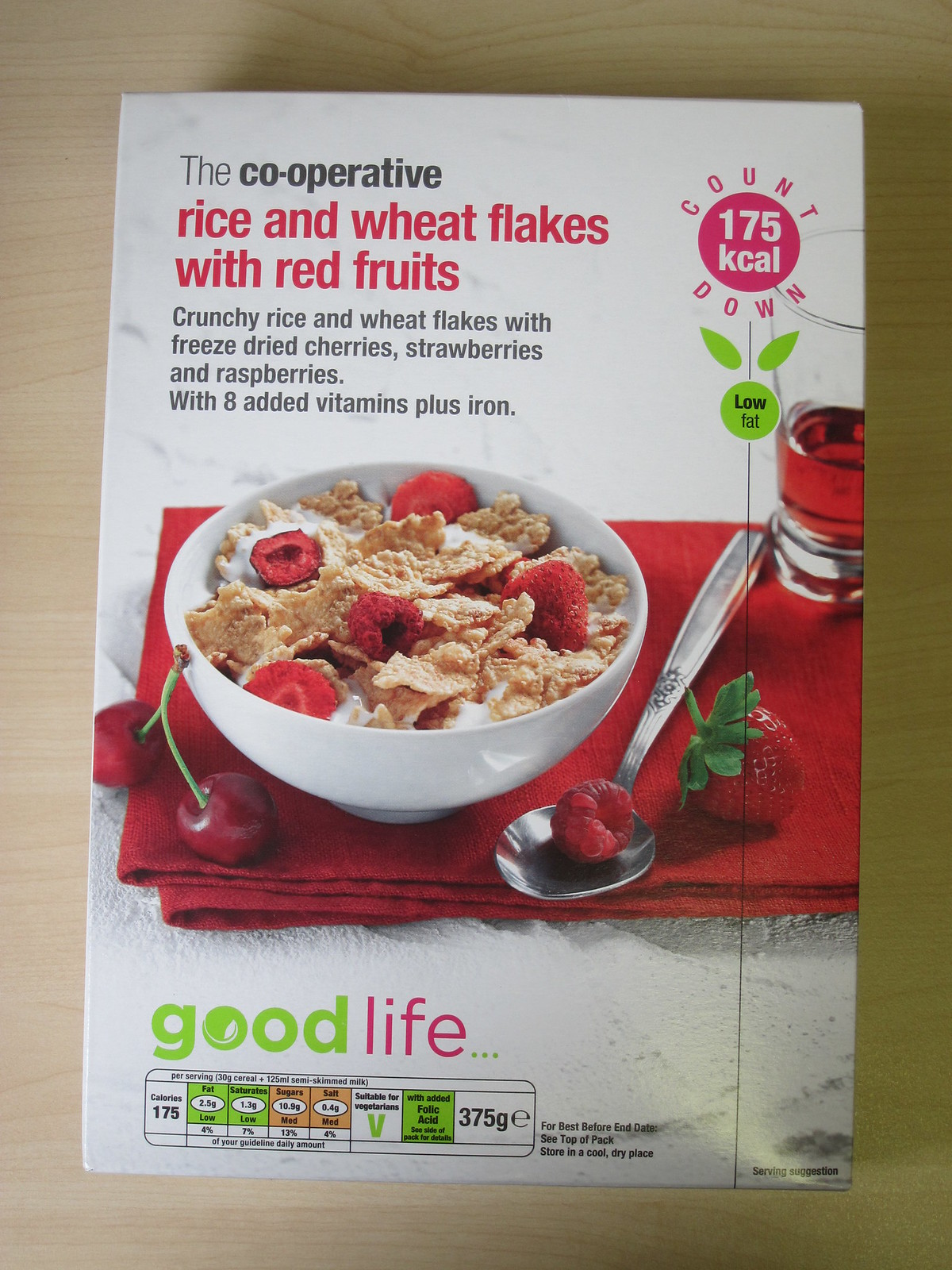The image depicts a cereal box laid flat on a light tan wooden table with visible grain. The background of the box is white, featuring a detailed photo in the center. The centerpiece of the photo is a white bowl filled with crunchy rice and wheat flakes, milk, and cut-up strawberries and raspberries. The bowl is placed on a red folded cloth, which also holds additional strawberries, a couple of cherries, a silver spoon with a raspberry on it, and a glass containing a brown beverage.

Text on the cereal box includes multiple pieces of information. In the top left corner, it reads: "The Cooperative Rice and Wheat Flakes with Red Fruits." Below that, in black text, it states: "Crunchy rice and wheat flakes with freeze-dried cherries, strawberries, and raspberries with eight added vitamins plus iron." The top right corner displays "175 Kcal" in a green circle, indicating it is low fat. The bottom left corner features "Good" in green and "Life" in red. At the very bottom, there is a section with detailed nutritional information.